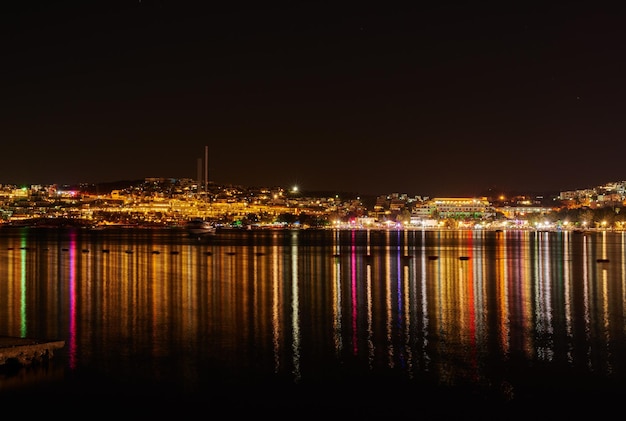This full-color nighttime photograph, taken from a vantage point in the harbor, captures a stunning cityscape against the black canvas of the night sky, devoid of stars or clouds. The rectangular image, notably free of borders, splits horizontally between the dark sky above and the calm water below, the latter occupying the entire lower half. The city, resting on slightly sloped hills and comprising various illuminated buildings, spans vertically between these halves. The myriad of city lights casts a vivid array of colors—whites, blues, purples, reds, oranges, pinks, hot pinks, neon greens, and yellows—onto the water, creating vertical streaks and a mesmerizing rainbow-like reflection that stretches across the harbor towards the photographer.